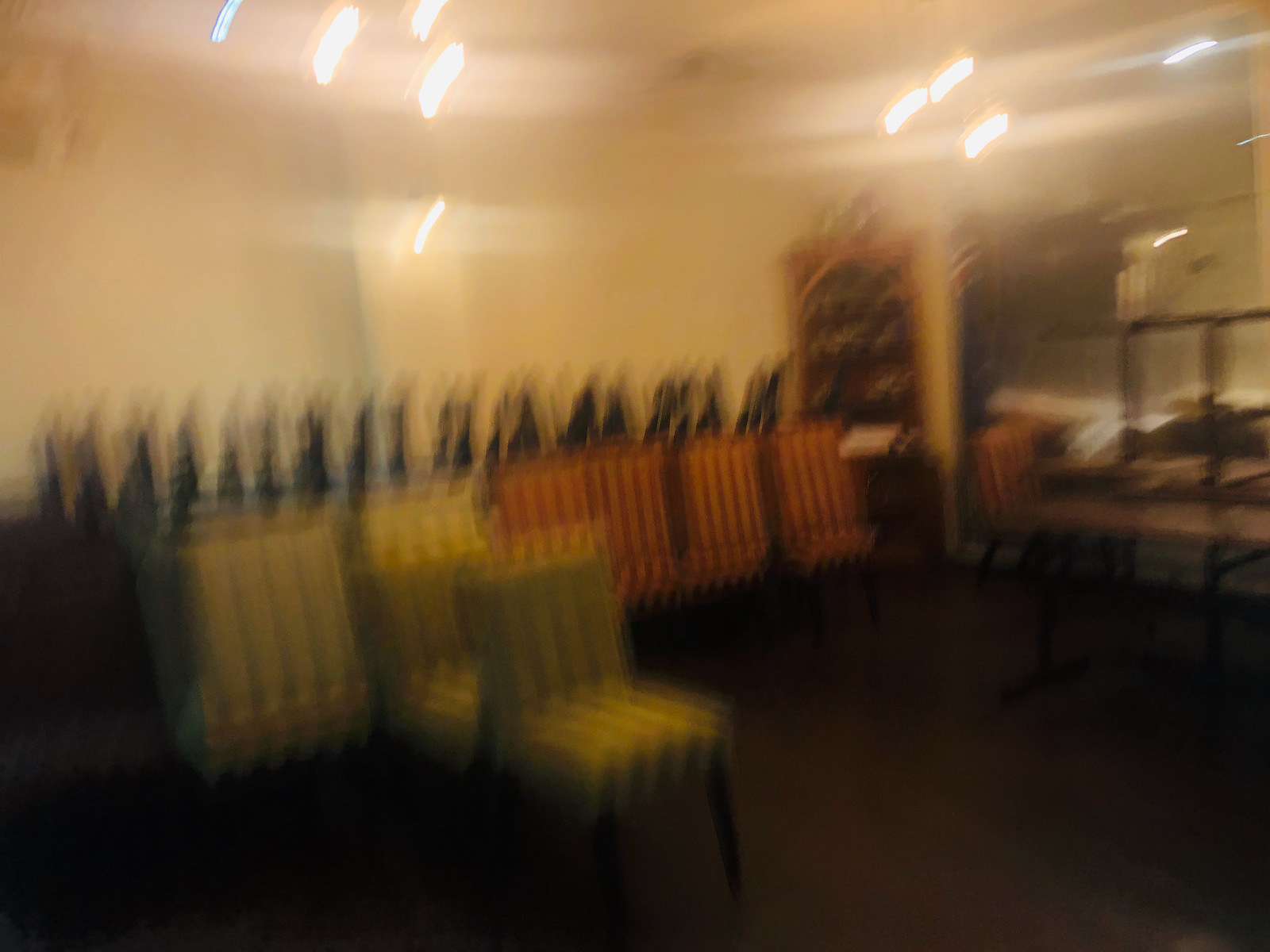The image is an extremely blurry and out-of-focus photograph of what appears to be a room, possibly a restaurant, banquet, or party venue. The image is wider than it is tall and exhibits considerable motion blur, with objects streaked and details hard to discern. In the room, there are numerous chairs either stacked or arranged in columns against an off-white wall with vertical stripes.

On the left side of the image, there are two chairs that appear to be standing upright. These chairs seem to be yellow with darker stripes, and they have darker, possibly brown legs. Close to these chairs, moving towards the right, you can see around four red chairs with lighter stripes and brown legs. Further to the right, closer to the middle and the right side of the image, more chairs are stacked in rows, possibly indicating they are stored this way.

The wall behind these chairs is off-white. There is mention of a conspicuous cabinet about two-thirds of the way over in the picture. This cabinet is only partially visible, with its details blurred and difficult to discern. Beyond this, there may be another wall or even a mirror giving a vague reflection.

Additionally, some elements like a table with black legs appear on the far right side of the image. The floor is brown, and the ceiling has a few lights that cast a blur across the scene. Overall, details in the room aside from the mentioned items are difficult to make out due to the blurriness of the image.